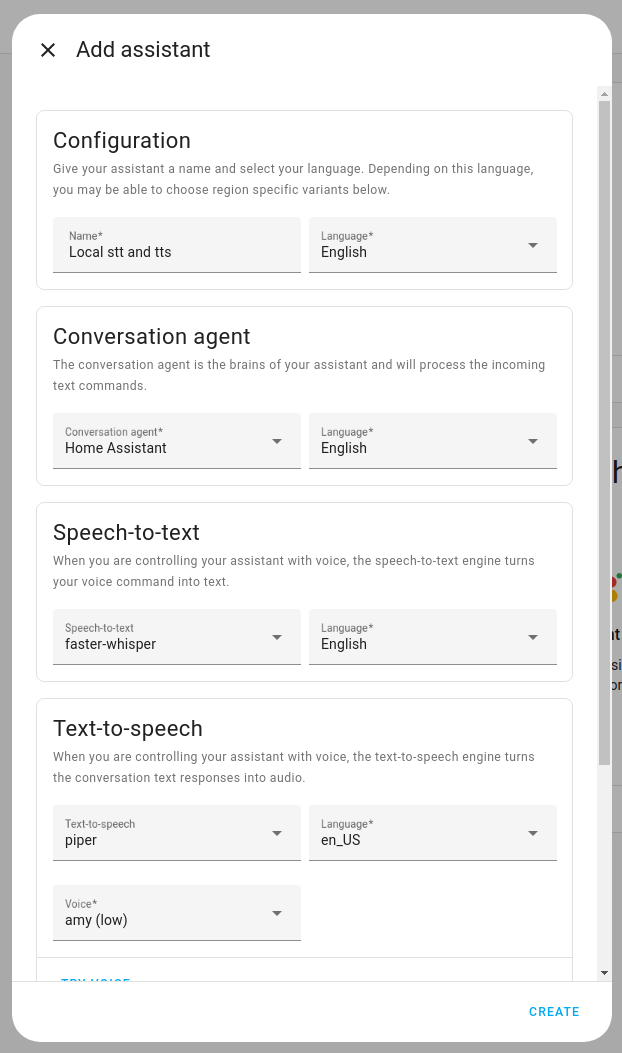This screenshot displays a detailed configuration menu for a text-to-speech and speech-to-text assistant setup. 

In the upper left corner, there is an "X" button for closing the menu. To the right, there is an option labeled "Add Assistant." Below that, the heading "Configuration" guides users to "Give your assistant a name and select your language. Depending on the language you choose, you may be able to select region-specific variants below."

The configuration sections are organized as follows:

1. **Name, Locale, STT, and TTS Settings:**
   - **Name**: Field for naming the assistant
   - **Locale**: Options for setting locale-based preferences
   - **Speech-to-Text (STT) Language**: Selected as English
   - **Text-to-Speech (TTS) Language**: Selected as English

2. **Conversation Agent Settings:**
   - The description emphasizes that the Conversation Agent processes incoming text commands, effectively serving as the "brains" of the assistant.
   - **Conversation Agent**: Home Assistant
   - **Language**: English

3. **Speech-to-Text Settings:**
   - Explanation that this engine converts voice commands into text for control via voice.
   - **Speech-to-Text Engine**: Fast Whisperer
   - **Language**: English

4. **Text-to-Speech Settings:**
   - Explanation that this engine converts conversation text responses into audio.
   - **Text-to-Speech Engine**: Piper
   - **Language**: EN_US
   - **Voice**: Amy Low

At the bottom right corner of the screen, there is a blue button labeled "Create" to finalize the setup.